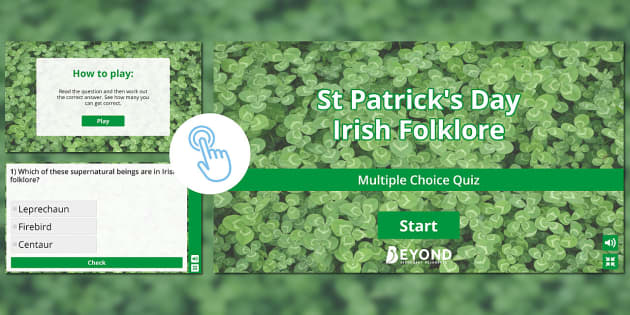The image is a promotional banner for a "St. Patrick's Day Irish Folklore Multiple Choice Quiz." The background is blurred, featuring a recurring clover pattern. Central to the image is clear signage with the quiz's title. Below this, there is a start button prominently displayed, with an emoji hand pointing at it to indicate where to begin. The image also includes a sample question that asks, "Which of these supernatural beings are in Irish folklore?" with the options: a. leprechaun, b. firebird, and c. centaur. Additionally, there's an indication of how to play the quiz within a white box in the top left corner, though the text here is fine and somewhat difficult to read. The name of the quiz's creator, possibly "beyond," is mentioned, with the letter B styled in an abstract pattern that makes it hard to decipher.